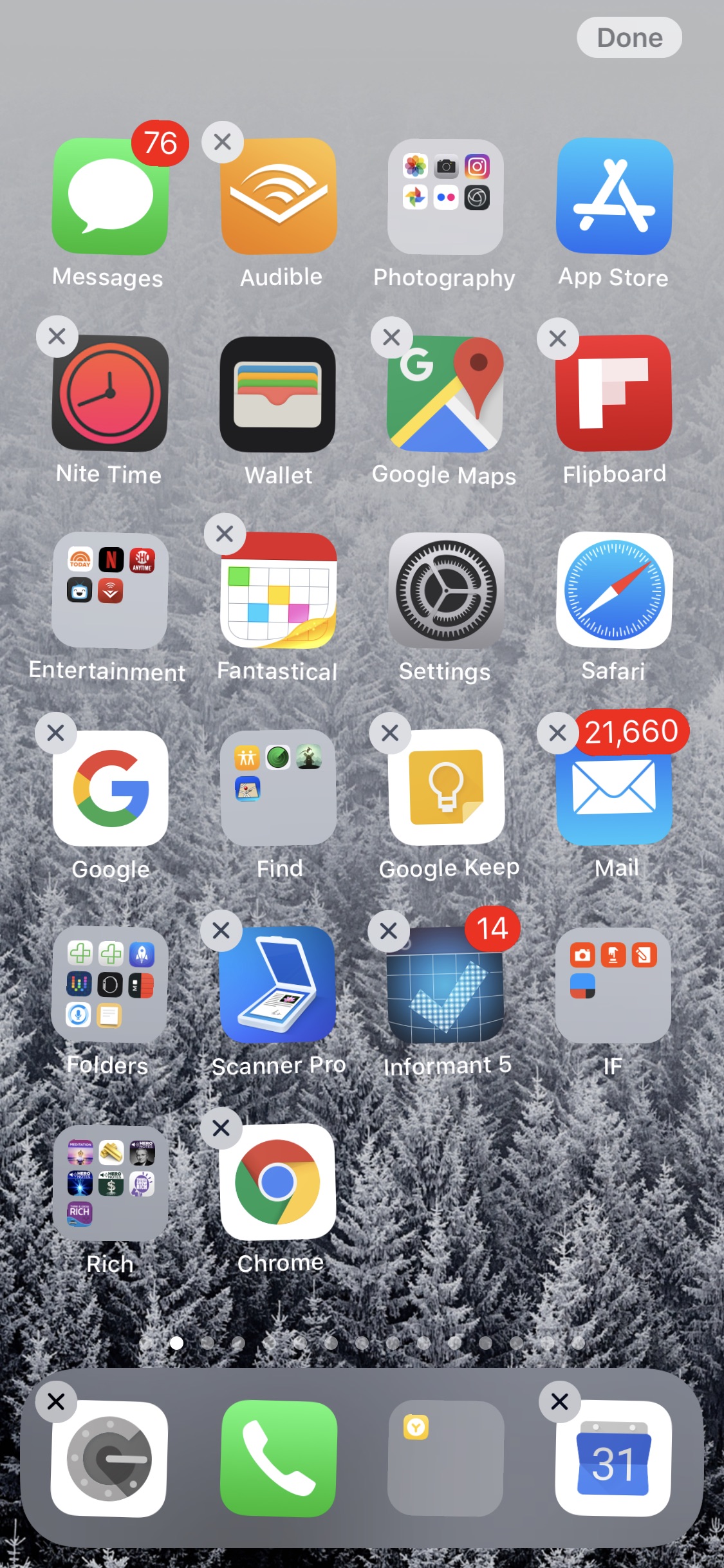The screenshot in question showcases an iPhone home screen with a gray background adorned with lovely evergreen trees at the bottom. It appears these trees might be snow-covered, though it's somewhat ambiguous. The apps are organized in several rows, each containing four apps:

1. **Top Row:**
   - Done (located on the far right)
   - Messages (indicating 76 unread messages)
   - Audible
   - Photography
   - App Store

2. **Second Row:**
   - Night Time (possibly NITE Time)
   - Wallet
   - Google Maps
   - Flipboard

3. **Third Row:**
   - Entertainment
   - Fantastical
   - Settings
   - Safari

4. **Fourth Row:**
   - Google
   - Find Google Keep
   - Mail (showing a staggering 21,660 unread emails)

5. **Fifth Row:**
   - Folders
   - Scanner Pro
   - Informant 5 (showing 14 notifications)
   - IF

6. **Sixth Row:**
   - Rich
   - Chrome

At the bottom of the screen, there are four additional icons whose details are as follows:
   - A gray circle in a white box
   - A green box with a phone icon
   - A gray box
   - A white box displaying the number "31," which likely indicates the date.

This meticulously organized home screen offers a glimpse into a user's array of frequently accessed applications.